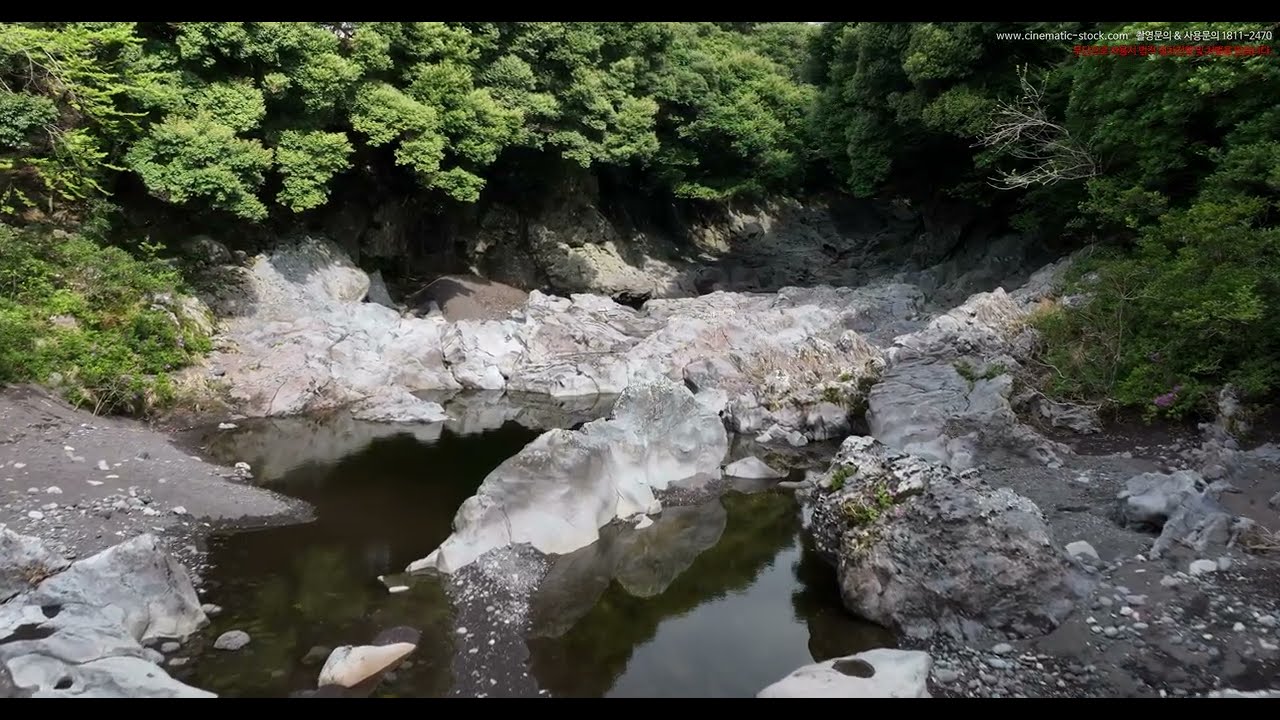The photograph depicts a tranquil creek set in a rugged, rocky landscape. The water, though dark with a greenish-brown hue due to reflections, remains clear enough to reveal the rocky bottom. The creek is bordered by numerous large, sharp, light gray and white stones, creating a stark contrast with the dark water. Surrounding the creek is a densely packed forest with scraggly green trees whose rich foliage reflects off the water, further enhancing its greenish tint. The scene extends into the distance, resembling a valley covered with rocks and pockets of dirt. In the upper right corner of the image, there is white lettering that reads "www.cinematic-stock.com," accompanied by some Asian characters and the numbers "1811-2470."